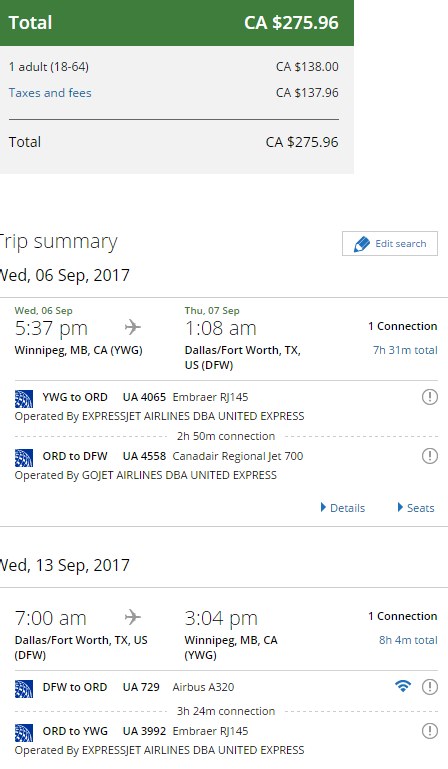This image appears to be a screenshot from a mobile phone displaying a detailed flight itinerary and cost breakdown. At the top, a green arrow icon highlights the total cost of the trip, which is $275.96 in Canadian dollars (CA). The breakdown indicates one adult traveler aged 18 to 64, with a base fare of CA $138.00 and additional taxes and fees amounting to CA $137.96.

The itinerary includes a "Trip Summary" section, detailing the departure and return flights:

**Departure:**
- Date: Wednesday, September 6, 2017
- Departure Time: 5:37 PM
- Departure Location: Winnipeg, MB, Canada
- Arrival Location: Dallas/Fort Worth, TX, USA
- Arrival Time: 1:08 AM (next day)
- Total Flight Time: 7 hours and 31 minutes
- Connection: 1

**Return:**
- Date: Wednesday, September 13, 2017
- Departure Time: 7:00 AM
- Departure Location: Dallas/Fort Worth, TX, USA
- Arrival Location: Winnipeg, MB, Canada
- Arrival Time: 3:04 PM
- Total Flight Time: 8 hours and 41 minutes
- Connection: 1

It is indicated that the traveler has a connecting flight identified by the airport code ORD (likely Chicago O'Hare International Airport). The layover time for this connection is 3 hours and 24 minutes before boarding flight UA-3992 to reach the final destination.